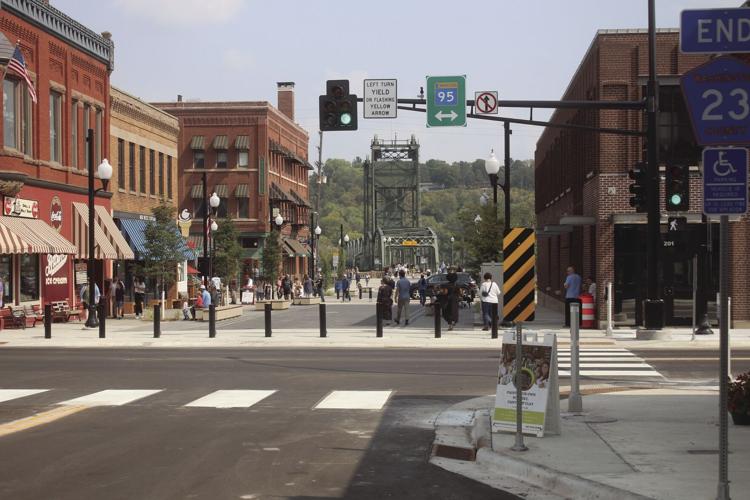This photograph captures a vibrant three-way intersection in a town likely in the United States, possibly at the end of Highway 23 and where Interstate 95 intersects. The view showcases a large plaza where the road ends and becomes a pedestrian-only zone, enhanced by planters, black poles, and barriers to prevent vehicular access. People are seen walking about, enjoying the day under a clear, blue sky that hints at spring or summer due to the leafy trees around. The intersection is adorned with a hanging stoplight and street signs. Surrounding the plaza are buildings that house commercial stores, some made from red brick and others from red stucco, with colorful awnings enhancing the scene. Off in the distance, a notable metal bridge extends, likely over a river, with a hill lush with trees rising in the backdrop. Prominent crosswalks connect the sidewalks and guide pedestrians through this lively urban space.